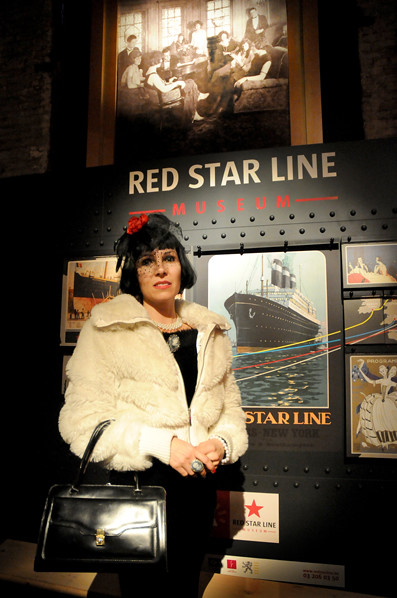A woman with light skin and a stylish, vintage look poses elegantly in front of a black wall at the Red Star Line Museum. The wall features white lettering at the top that reads "Red Star Line Museum" and is decorated with various vintage photographs, including images of ships and groups of people. She is dressed in a white fur coat that reaches her waist, with a black dress underneath. She accessorizes with a diamond necklace, a black handbag with a shiny silver clasp, and a black hat adorned with red flowers and a slight veil. Her short bob of black hair frames her face, showing off her full makeup and red lipstick. She stands with her hands clasped in front of her waist, her right arm looped around the handbag’s handle, with a ring on her index finger, and she gazes forward toward the camera.